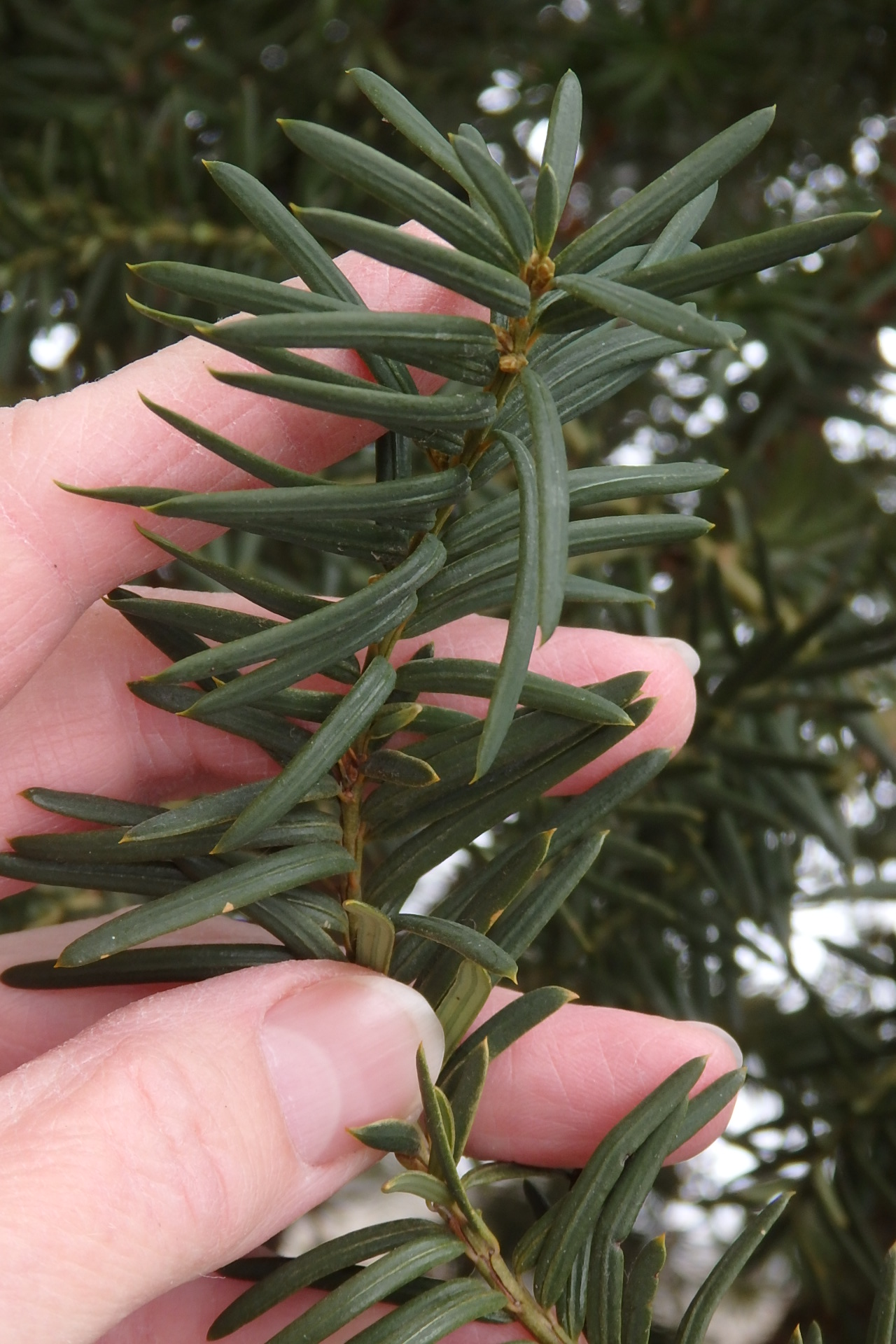The image is a highly detailed and close-up nature photograph of a Caucasian person's hand holding a delicate branch of an evergreen plant, possibly Japanese Yew. The hand is positioned in such a way that the thumb supports one end of the branch while the other fingers cradle the tip, showcasing the plant's health. The branch, a thin brown stick, features blade-like dark green leaves that are straight and stiff, radiating in all directions. The background hints at a wintry setting, with glimpses of snow visible through the branches of what appears to be a pine tree, along with other similar trees. This juxtaposition emphasizes the plant's robust green color against the colder, snow-dusted scenery.